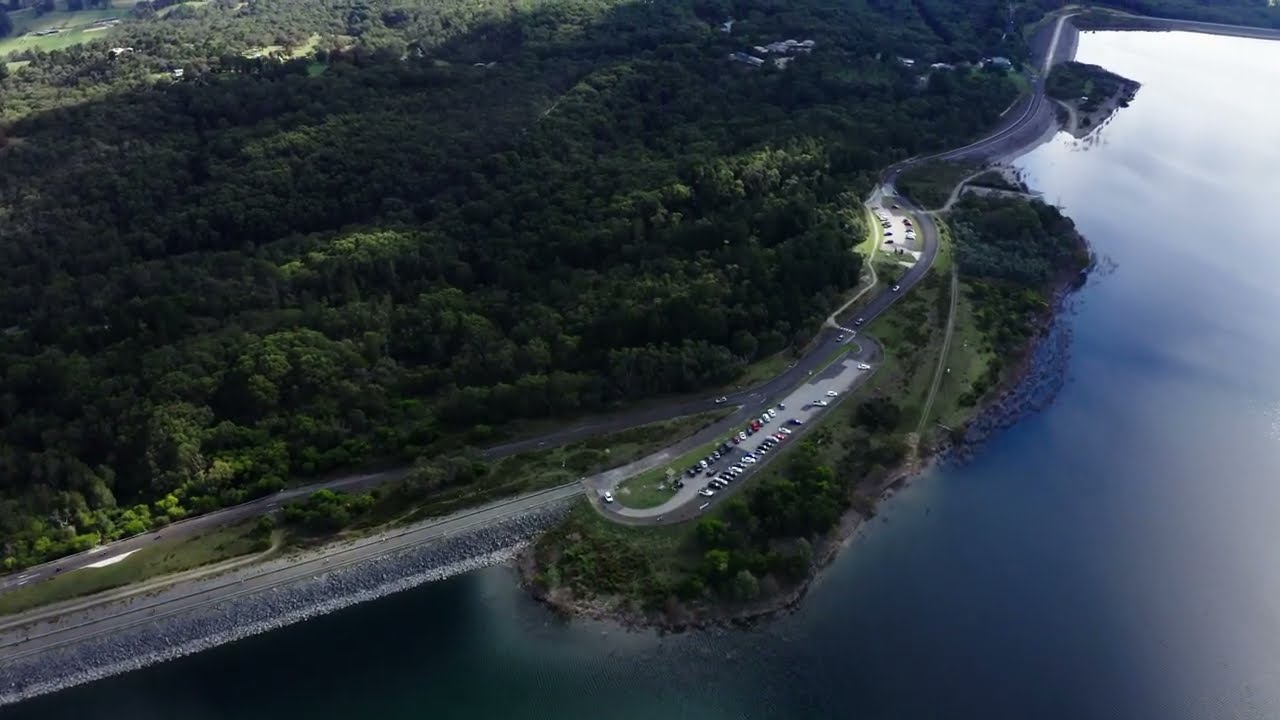This aerial view captures a vast, lush forest occupying approximately 60% of the left side of the image. The dense, green trees blanket a landscape of rolling hills, whose elevation is difficult to discern. To the right, a large body of water, possibly a major lake or a section of ocean, reflects a navy blue hue with light glinting off its surface in the top right corner. The shoreline is rugged with an abundance of rocks meeting the water. Running parallel to the edge of the forest is a winding road, adjacent to a parking lot filled with numerous cars that appear tiny from this high vantage point. While the cars and outlines of people resemble small ants due to the distance, the scene is completed by the peaceful interaction of land, water, and human presence.